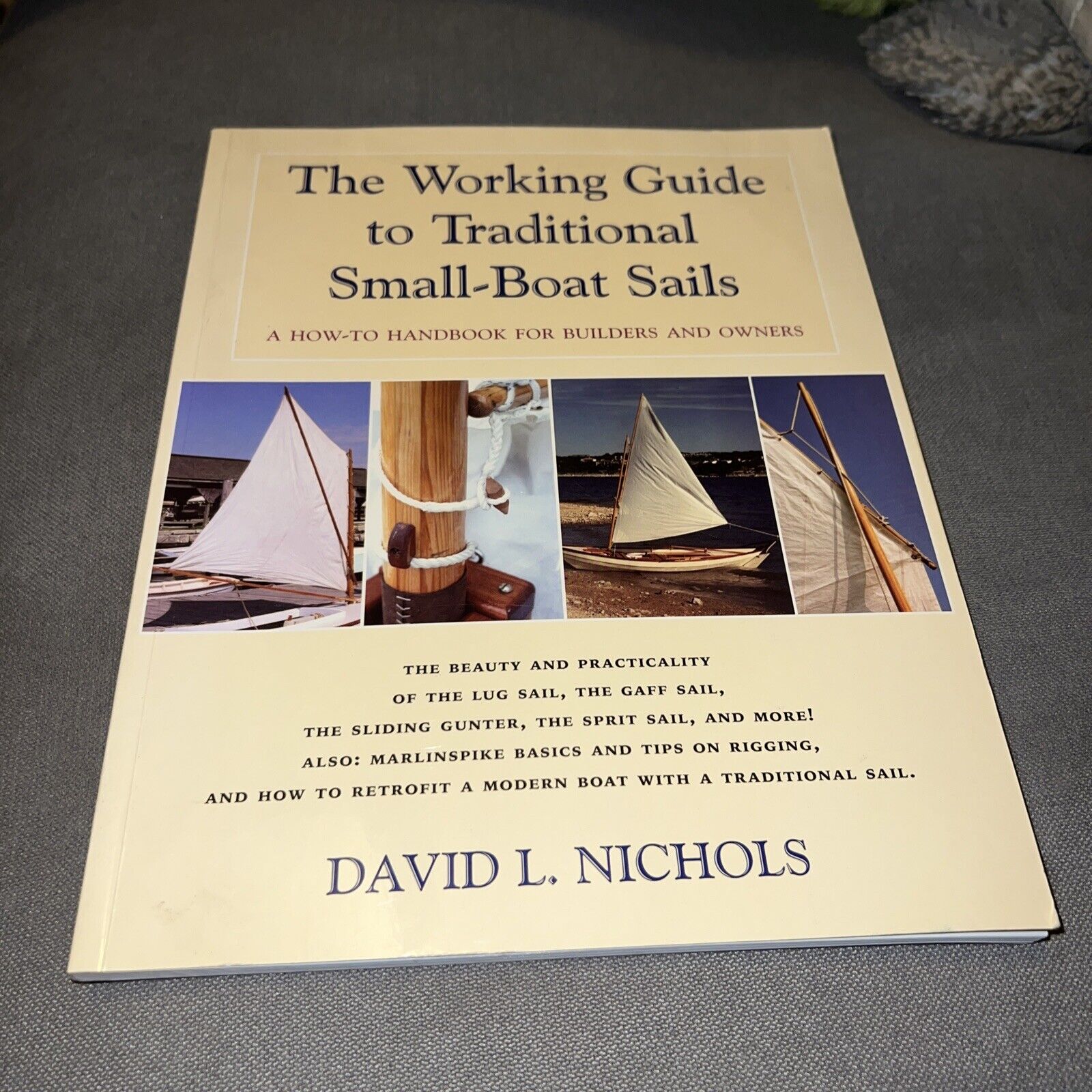This photograph features a beige-colored, soft-cover book titled "The Working Guide to Traditional Small Boat Sails: A How-To Handbook for Builders and Owners" by David L. Nichols. The text on the cover is prominently displayed in blue and black. At the center of the cover, there are four sub-sectional images. These images include a close-up of a sail, detailed knots and rope work on wooden structures of the boat, a sailboat docked at shore, and another intricate section of the sail itself. Beneath these images is additional text that reads: "The Beauty and Practicality of the Lug Sail, the Gaff Sail, the Sliding Gunter, the Sprit Sail, and more. Also, Marlin Spike Basics and Tips on Rigging and How to Retrofit a Modern Boat with a Traditional Sail." The book lies on a gray surface, capturing both its detailed content and the nuanced aesthetics of traditional small boat sails.